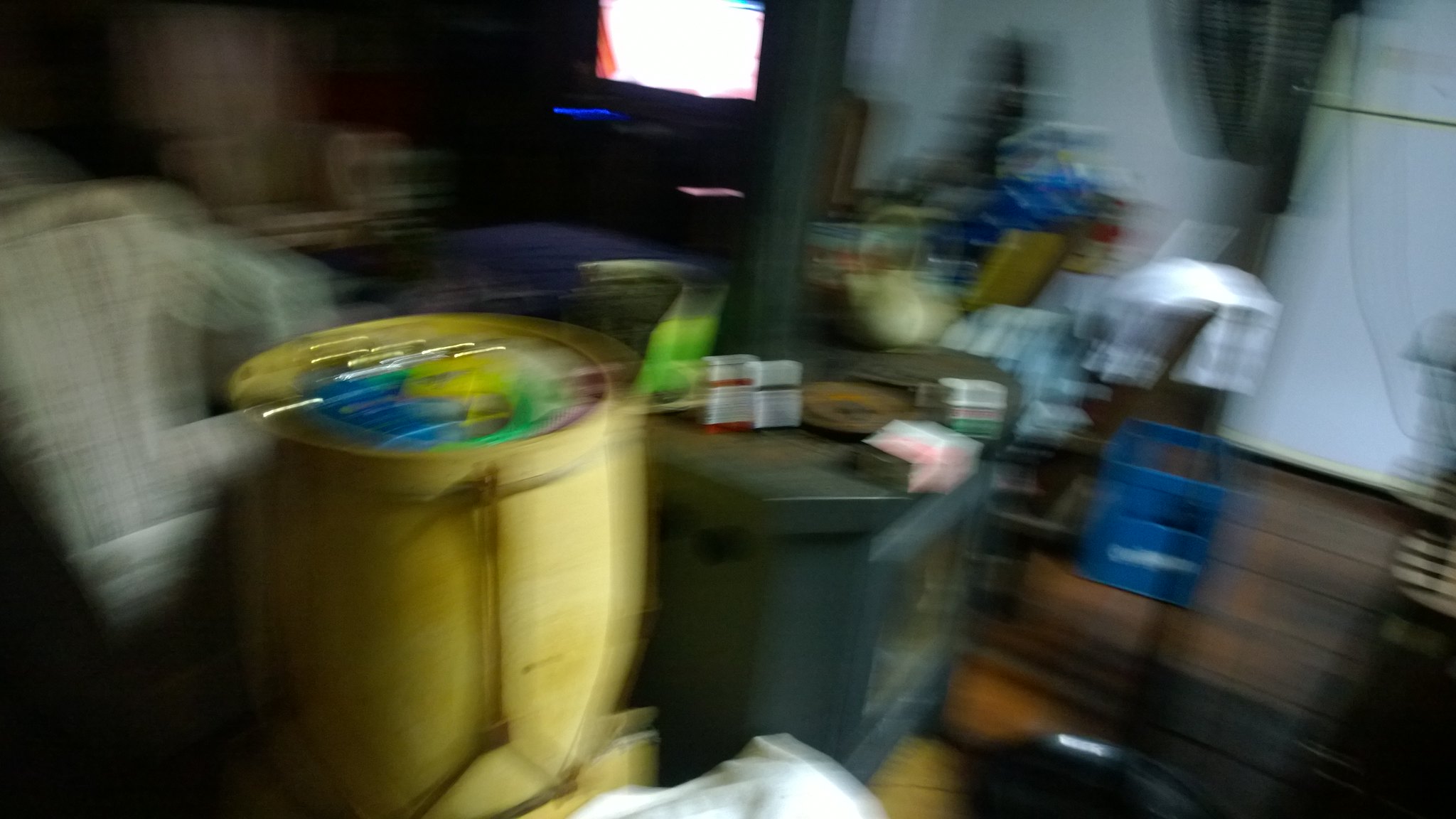In this photograph, we see a room that is very out-of-focus and riddled with motion blur, suggesting the photographer was moving while taking the shot. The room has a somewhat cluttered appearance. On the left-hand side, a prominent yellow container or possibly a 55-gallon drum stands out. On top of or near the yellow drum is an assortment of items that have blue, green, gold, and a hint of red colors. Right next to this yellow container appears to be an octagonally shaped wood stove with angled edges and a door that has a transparent glass pane. A duct extends from this stove toward the ceiling. To the right of this setup, there's a green table with several small white boxes on top. In the distant background, there's a television screen emanating a glow, indicating it's turned on, adding a faint light to the scene. Scattered around the room, particularly towards the back, are various items, which include blue and white carton containers, all resting on a dark, wooden floor.